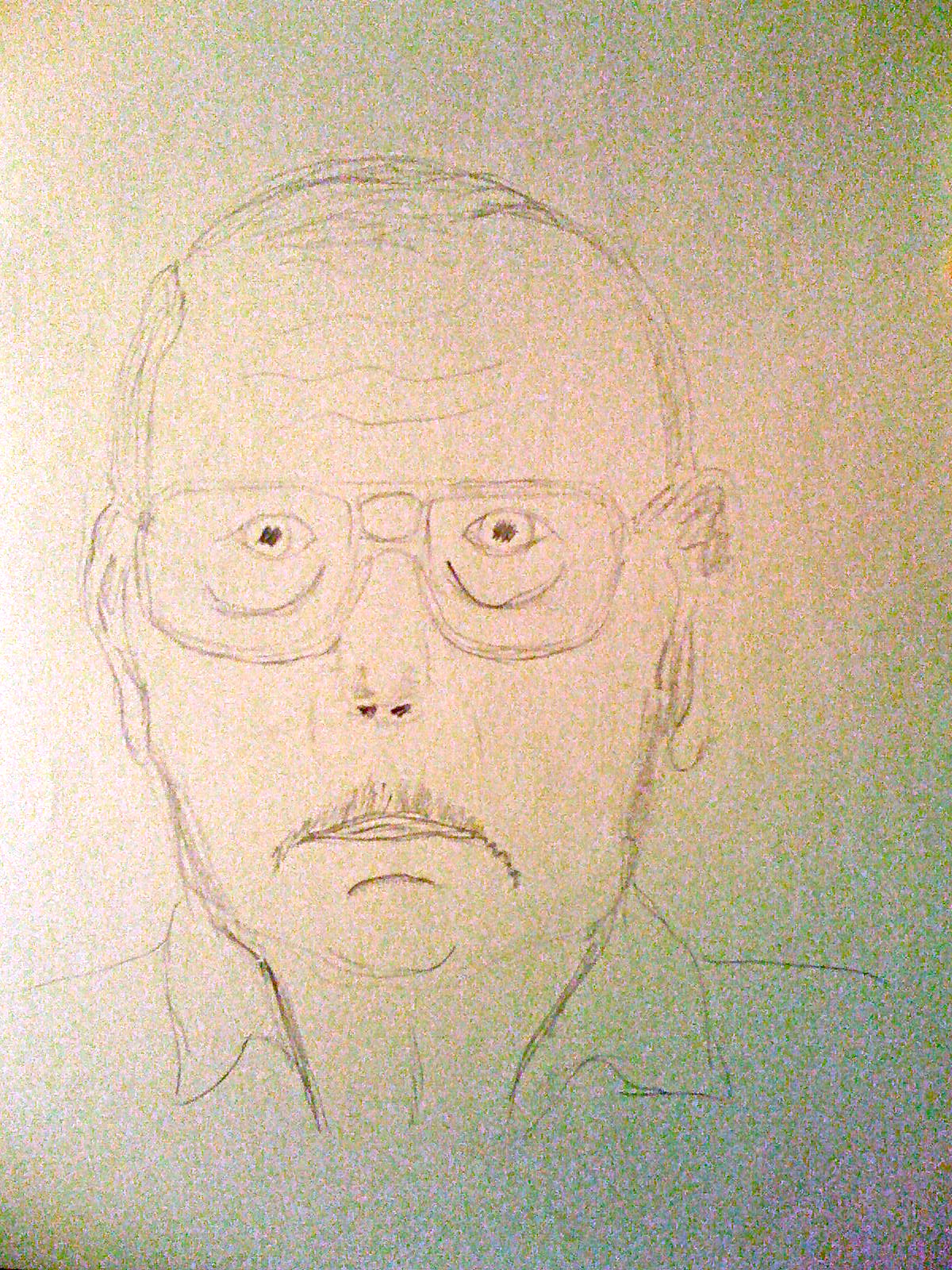This image captures a detailed pencil sketch of an elderly man, drawn on a greenish-brown sheet of paper. The man, who is predominantly bald but has a bit of hair combed over the top, is shown with prominent facial features. He wears large, horn-rimmed glasses and has intense, dark pupils within wide, staring eyes, giving him a somewhat unsettling expression. His forehead is marked with multiple lines, and there are additional curved lines beneath his eyes. His thin mustache rests just above his upper lip, with the rest of his face clean-shaven. The sketch includes a detailed depiction of his facial structure, including ears and a rounded chin, and the man also wears a collared shirt, represented by two visible collars on either side of his neck.